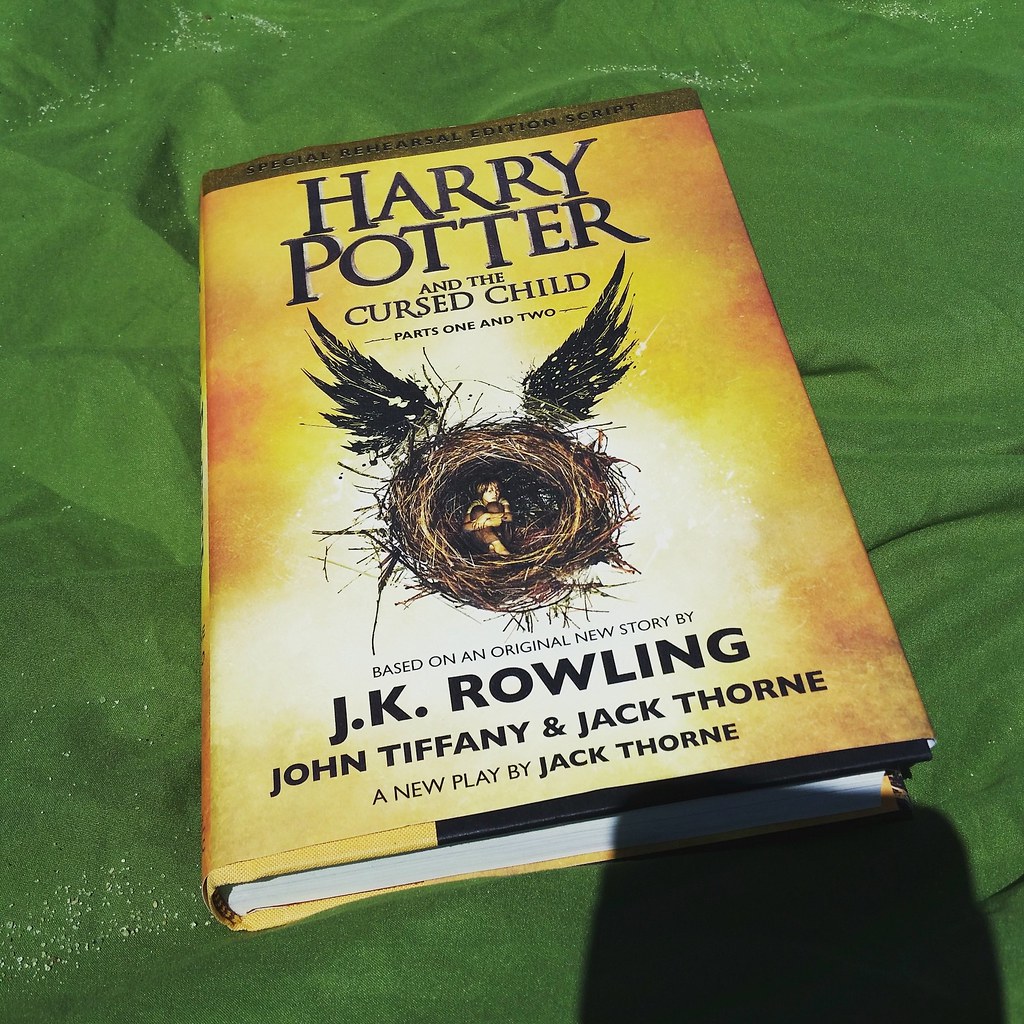In this indoor image, a single hardcover book titled "Harry Potter and the Cursed Child, Parts 1 & 2," based on an original new story by J.K. Rowling, John Tiffany, and Jack Thorne, and written as a new play by Jack Thorne, takes center stage. The book is positioned diagonally in the middle of the photo, resting on a green fabric that appears to be a wrinkled sheet or blanket. The cover of the book features an orange and yellow gradient background with an illustration of a bird’s nest containing a young child from which wings sprout on the sides. The title and the authors' names are prominently displayed, with the "Harry Potter" logo appearing in dark blue and the names J.K. Rowling, John Tiffany, and Jack Thorne in black. There are small crumbs or specks visible on the fabric, and a shadow—presumably from the smartphone being used to take the picture—can be seen in the bottom right corner of the image, adding a casual, candid element to the scene.